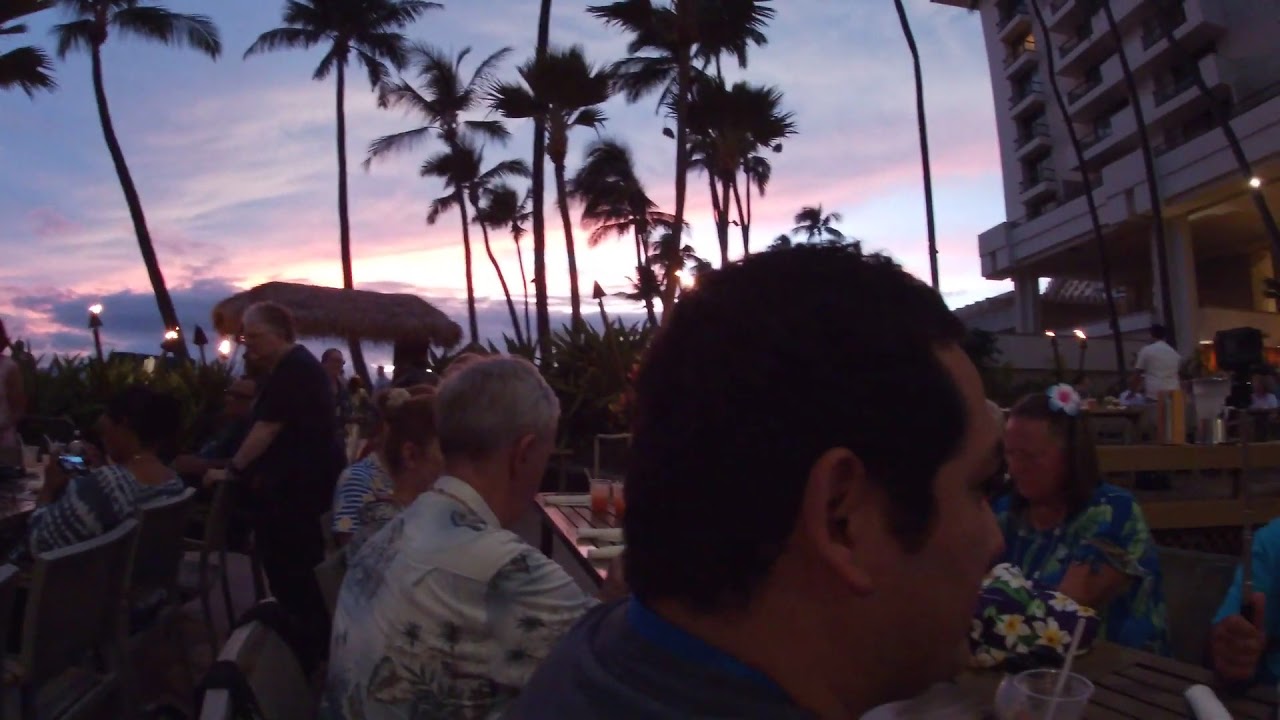The image depicts a dimly lit, slightly blurry scene at an outdoor restaurant, likely part of a hotel at a beach resort. Patrons, many dressed in Hawaiian-style floral shirts, are seated at long tables, engaged in dining and conversation. A woman on the right, notably wearing glasses and a white flower with a red center in her hair, stands out among the guests. Tiki torches punctuate the evening ambiance with their warm glow, as palm trees sway gently in the background. The horizon reveals a striking sunset, with purplish, dark gray clouds accented by rosy pinks and peaches, suggesting the last light of day. To the right, above the dining area, a hotel structure with multiple floors is partially visible, adding to the overall tropical atmosphere.